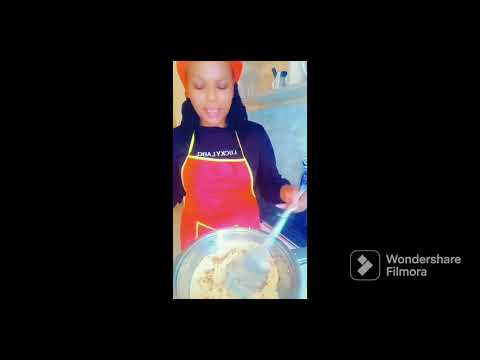The image is set within a black border that features the text "Wondershare Filmora" in white on the lower right corner, accompanied by a logo consisting of a square and a backwards L-shaped figure. At the center of the image, there's an African American woman with partially visible orange or bright red hair, seemingly wearing a head accessory that resembles a turban. She is dressed in a navy blue hoodie with indiscernible print and a vivid red apron accented with yellow straps, piping, and a pocket trim. The woman appears to be stirring or whisking something in a silver pot or mixing bowl, which contains a foamy tan-colored mixture, using a circular or spoon-like utensil. Her head is slightly tilted downwards, focusing on her cooking task. The image is in portrait orientation and appears to be a low-quality, possibly screen-captured, snippet, suggesting it might be from a video, potentially a TikTok clip.